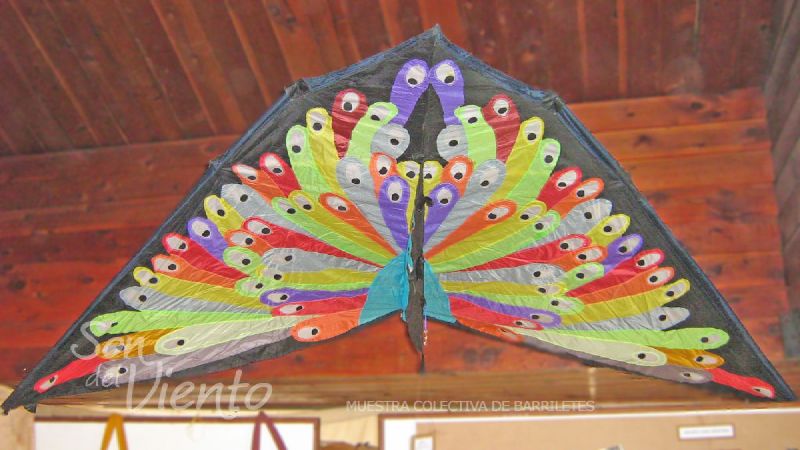The photograph showcases an ornate, triangular-shaped kite with a vibrant, multicolored design that mimics the appearance of peacock feathers. The kite, primarily black with a blue trim, features worm-like shapes in a spectrum of rainbow colors—red, orange, yellow, green, blue, purple, white, and more. Each "feather" emanates from the lower center part of the kite and is marked by a white dot with a black center, resembling eyes. 

The kite is positioned on a dark-stained, rustic wide-plank wooden floor, leaning slightly against the similarly dark wooden back wall, creating a cozy, rustic setting. Overlaying the image is text that includes "San Del Viento" and "Muestra Colectiva de Berroletes," suggesting it might be part of a promotional or artistic display, potentially from a foreign country. The colorful, eye-catching design fills every conceivable space, making the kite the compelling focal point of the image, against the warm, wooden backdrop that could be inside a cabin or a house.